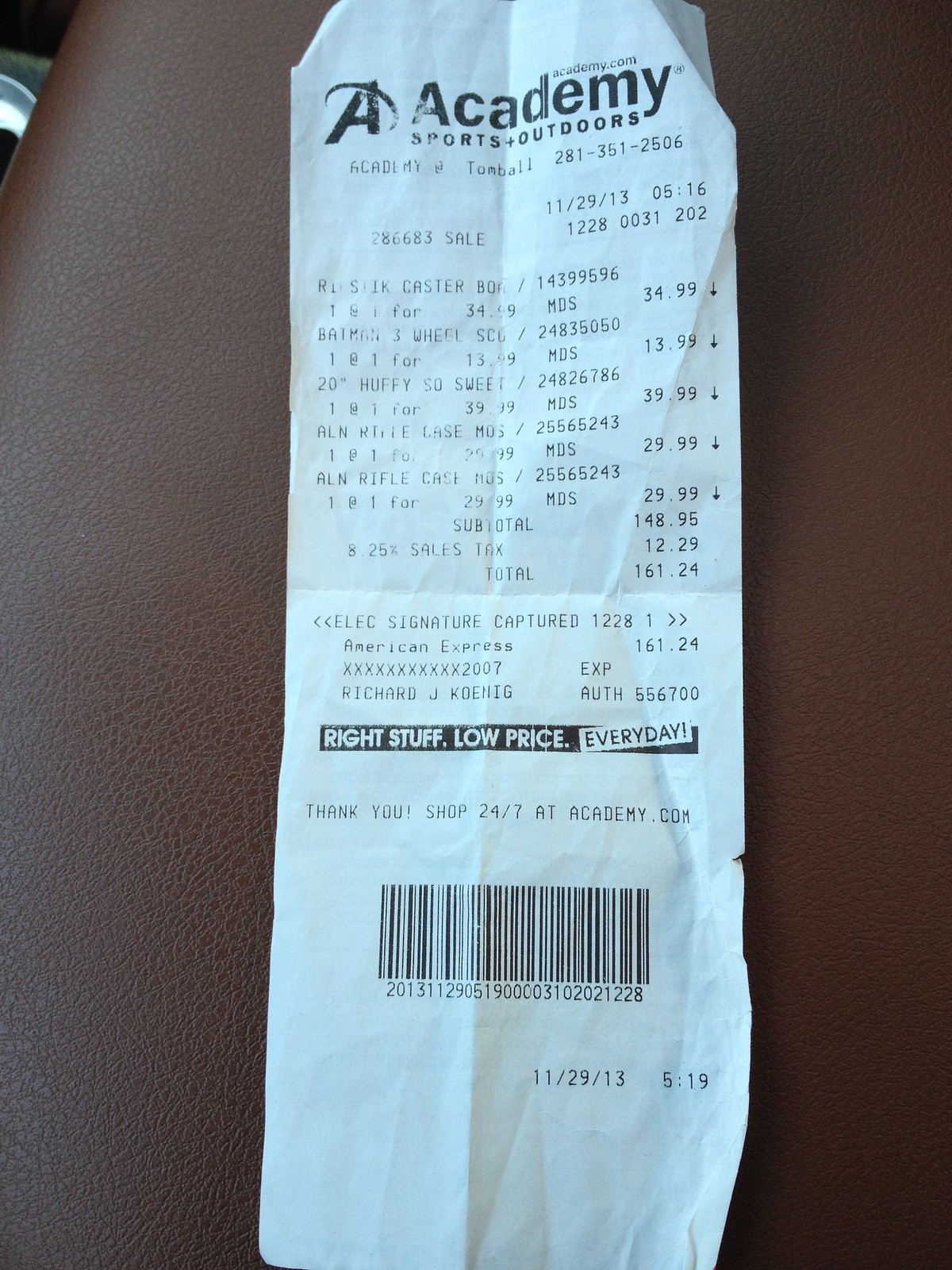The image captures a slightly faded and crinkled receipt resting on a brown leather chair. The receipt is from Academy Sports + Outdoors. At the top, it lists the store's phone number, followed by the date "11-29-13" and the time "6:16." Below that is a sale ID number. The receipt details the purchase of five items: the first priced at $34.99, the second at $13.99, the third at $39.99, and the last two items each at $29.99, summing up to a subtotal of $148.96. With an additional sales tax of $12.29, the grand total comes to $161.24. The payment was made using an American Express card, displaying only the last four digits: 2007, and under the name Richard J. Koenig. An authorization number is listed, followed by a thank you note and a prompt to shop online at academy.com. At the very bottom, there is a barcode along with a series of numbers, and the date "11-29-13" is reiterated.